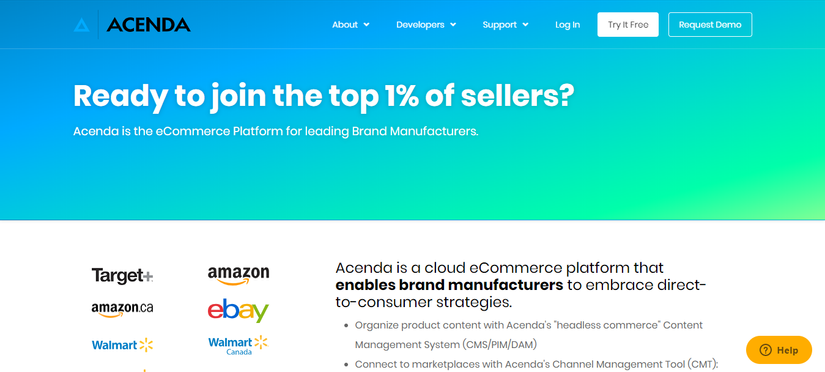This image is a screenshot of an e-commerce platform's landing page, divided into two distinct sections. 

The top section features a gradient blue rectangle that transitions from green at the bottom right to blue at the top left. Overlaying this gradient is the company's logo, "Ascendia," displayed both as text and a blue emblem in the top left. Positioned to the right of the logo are clickable columns labeled "About," "Developers," "Support," and "Login." Further to the right are two buttons: "Try It For You" and "Request Demo." Dominating the center of this section in large, bold text is a promotional message: "Ready to join the top 1% of sellers? Ascendia is the e-commerce platform for leading brand manufacturers," which seems to be an advertisement encouraging users to engage with Ascendia's services.

The bottom section of the image contrasts with a white background. On the right side, black text reads: "Ascendia is an e-commerce platform that enables brand manufacturers to embrace direct-to-consumer strategies," followed by additional supplementary text. Adjacent to this text on the left are logos of prominent companies such as Target, Amazon, eBay, and Walmart, likely indicating these firms as Ascendia's partners. Nestled to the side of the descriptive text is a small, pill-shaped help icon designed to assist users navigating the website.